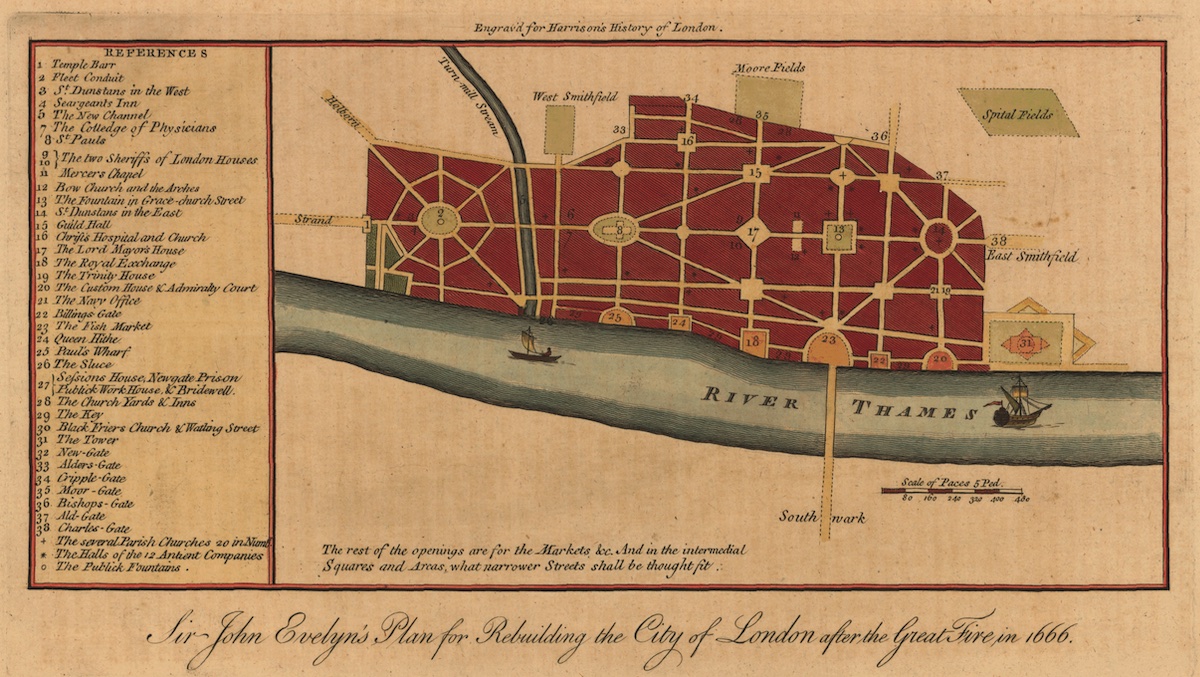This detailed image is an antique, hand-drawn map on faded orange or light tan paper, depicting Sir John Evelyn's Plan for Rebuilding the City of London after the Great Fire in 1666. It features an older, swooping cursive script in black font. Central to the map is the River Thames, illustrated in bluish-gray, with two ships drawn in for illustrative purposes. The main city plot is highlighted in red, with yellow indicating streets and numbered sections representing various planned buildings, such as the Royal Exchange (number 18) and Guild Hall (number 15). On the left side, there is a reference guide numbered from 1 to 38, detailing the significance of each section. The intricate detail, antique style, and historic context make this map a fascinating artifact representing post-fire city planning in London.